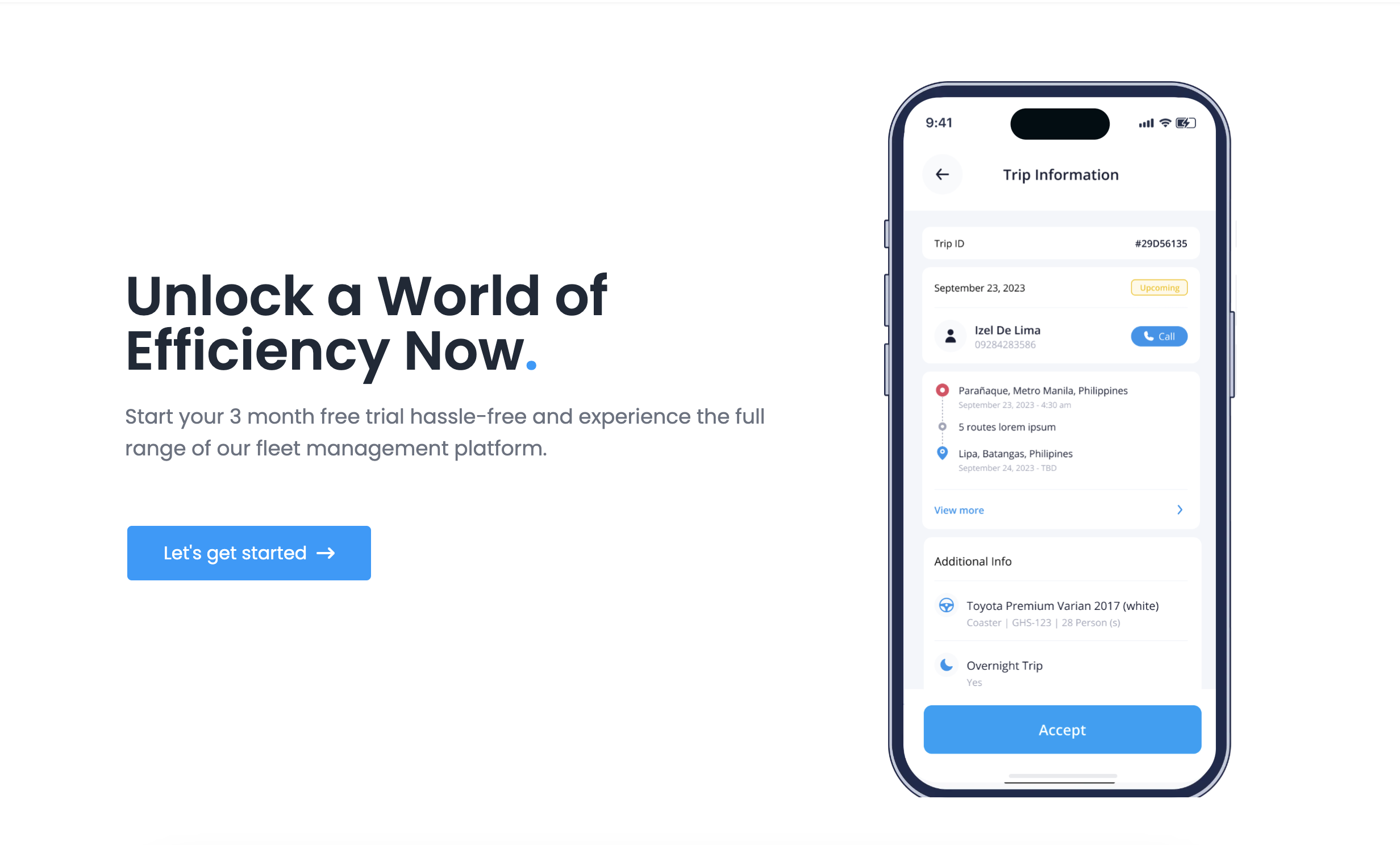This advertisement features a minimalistic design with a white background. The layout is divided into two sections. On the left, constituting two-thirds of the ad, there is a stark white space with centered text in bold black letters that read, "In a world of efficiency now." A small blue dot punctuates the statement. Below this, in gray text, the ad encourages viewers to "Start your three-month free trial, hassle-free, and experience the full range of our fleet management platform." Directly beneath this invitation, a blue button with white text urges viewers to act, stating, "Let's get started."

To the right, occupying the remaining third of the ad, is an image of a smartphone displaying the app's interface. The phone's status bar indicates the time as 9:41, with four signal bars and approximately half of the battery life remaining. The app screen is centered on trip information with a back arrow for navigation. The screen features a variety of details:
- A "Trip ID" consisting of a series of numbers, set against a white background.
- The date "September 23rd, 2023," accompanied by a yellow icon that is indistinguishable against the white background.
- An icon representing a person, with the name "Isel De Lima" beside it, although parts of this section are blurred out.
- A blue button labeled for call functionality, indicating that users can contact someone regarding their trip. Additional trip-related information is listed below this primary data.

This comprehensive and visually clean advertisement effectively showcases the key features of the fleet management platform, providing a clear call-to-action for potential users.